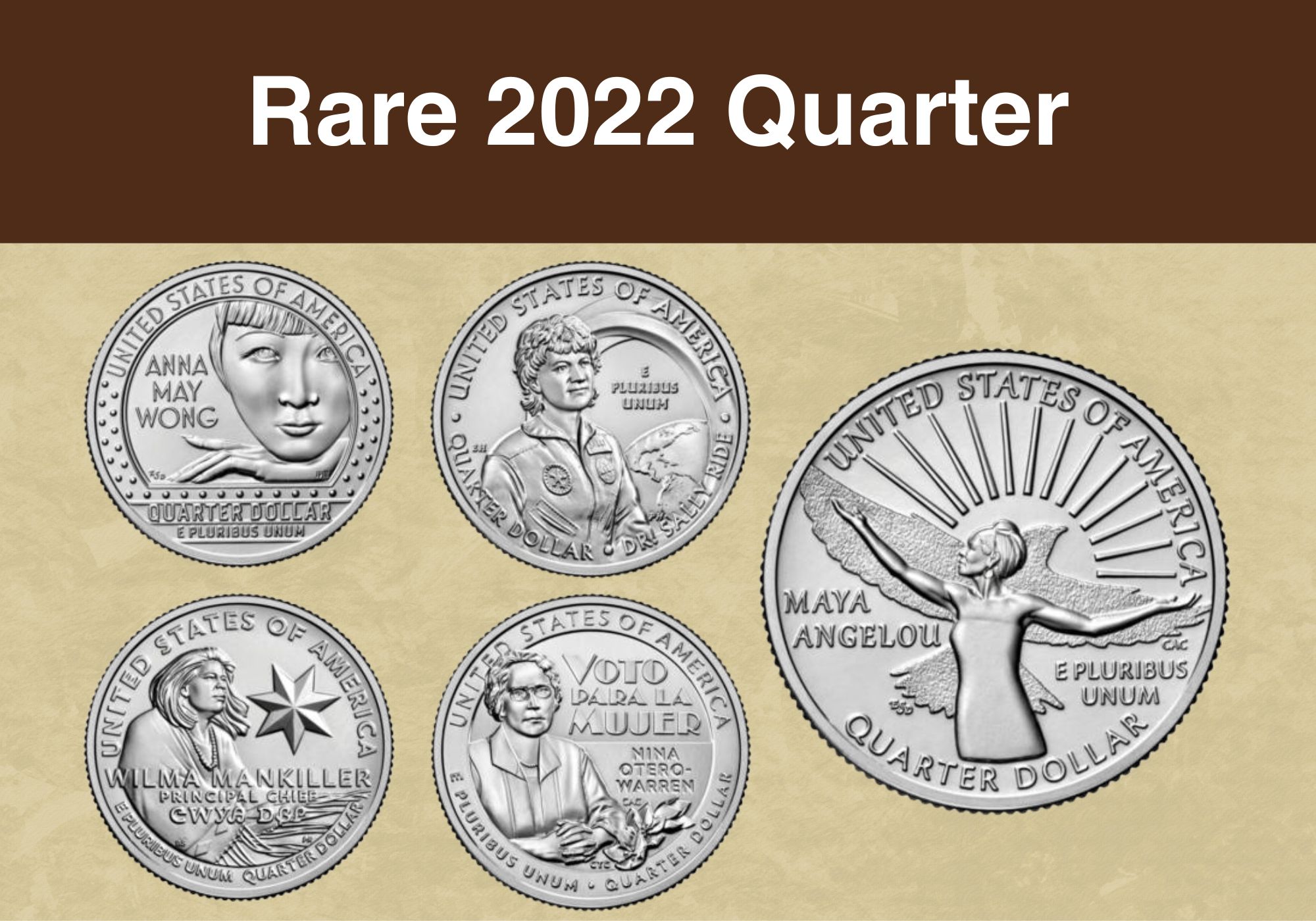The image is a detailed promotional illustration of five rare quarter dollars from 2022, set against a beige background. The top of the image features the bold white text "Rare 2022 Quarter" on a dark brown stripe. Below, displayed on the beige background, are five distinctive quarter designs, each depicting historic women. Positioned from left to right, the first four quarters are smaller, while the fifth, on the far right, is a larger image. The quarters feature the following notable women: Maya Angelou with her arms outstretched, Anna Mae Wong resting her chin on her hand, Dr. Sally Ride in her astronaut uniform, Wilma Mankiller seated next to a star emblem, and Nina Otero-Warren depicted sitting with her hands folded. All quarters are inscribed with "United States of America" and "E Pluribus Unum." The illustration serves as a mock-up of these rare quarter designs, highlighting their unique commemorative nature.